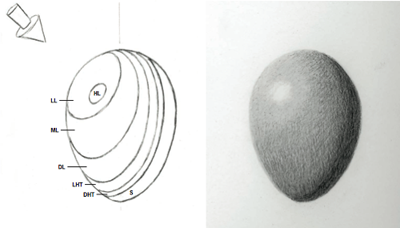The image in landscape mode consists of two side-by-side visuals, with the left side displaying a detailed drawing and the right showing a corresponding photograph. The photograph on the right showcases a spherical object, resembling a top shell or a stone, set against a dark gray background. The object is flat on the bottom and round on top, with its shaded areas transitioning from light to dark gray. 

On the left, the drawing replicates the photographed object and includes multiple concentric circles with annotations. An arrow points from the top-left corner towards these circles, which increase in size. Each circle or section is labeled with initials, indicating different measurements or layers: HL (innermost), LL, ML, DL, LHT, DHT, and S (outermost). The drawing highlights varied aspects of shading and lighting on the object, suggesting instructional elements on how to illustrate or analyze the layered structure and textures effectively.